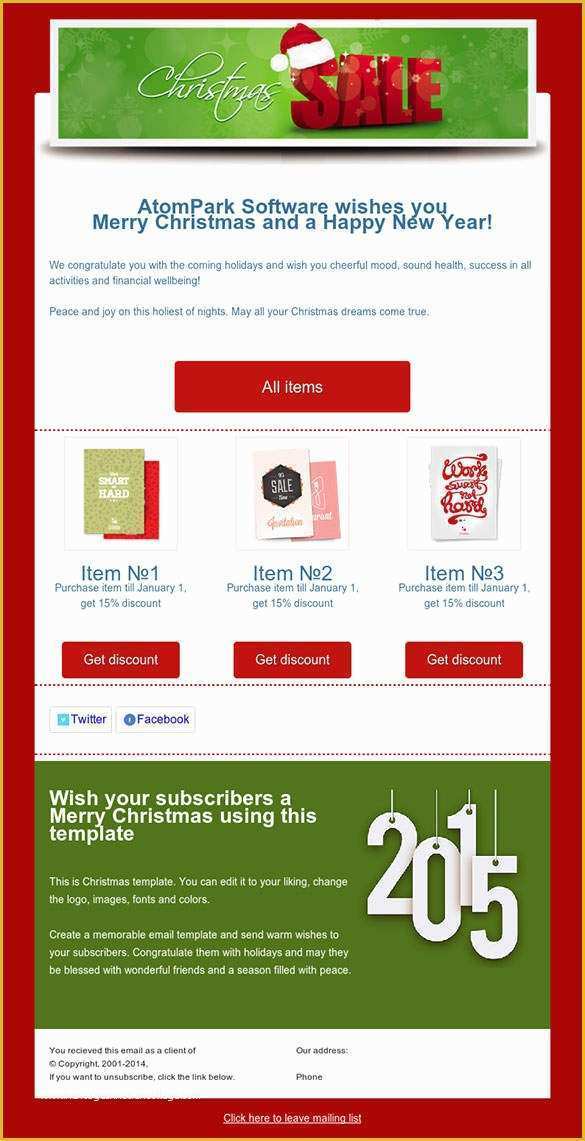This is a detailed screenshot of a festive website. The background is a vivid red, and at the very top, there's a banner designed as a white-outlined rectangle. In the center of this banner is a green graphic dotted with white spots, resembling snowflakes. In elegant white cursive font, the word "Christmas" is displayed, adjacent to large, red bubble letters spelling "SAIL." These letters are three-dimensional, highlighted with black shadows, and the "S" in "SAIL" is adorned with a Santa hat.

Beneath the banner, there's a prominent white square. Inside it, blue text reads: "Adam Park Software wishes you a Merry Christmas and a Happy New Year. We congratulate you on the coming holiday and hope and wish you a cheerful mood, sound health, success in activities, financial well-being, peace, and joy on this holiest of nights. May all your Christmas dreams come true."

Further down, a red rectangle with white font states, "ALL ITEMS." Below this is another white rectangle featuring three graphics that appear to be greeting cards. While the text on these cards is illegible, each card is labeled respectively as "Item Number One," "Item Number Two," and "Item Number Three."